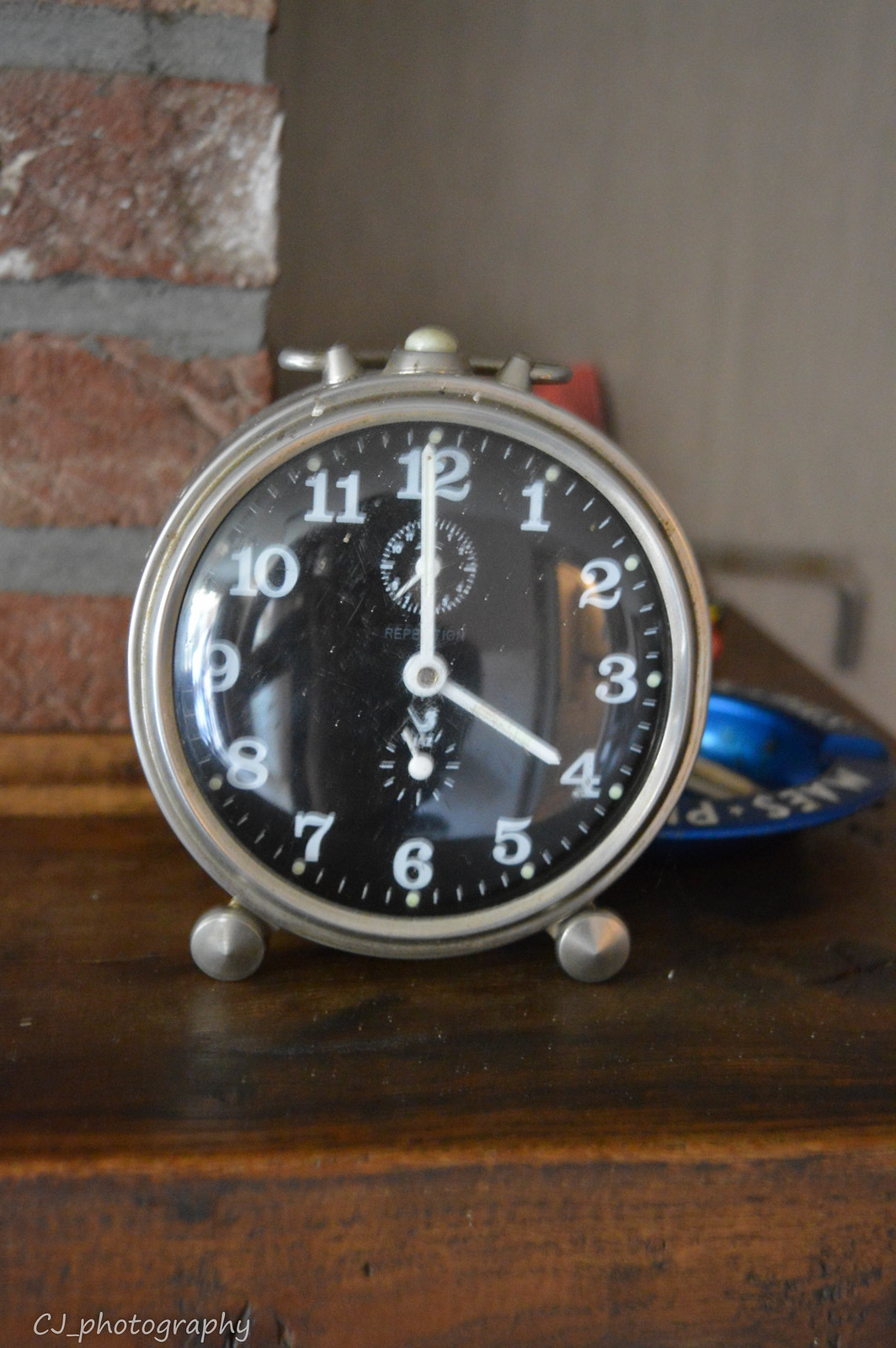The photograph captures a round, brushed silver analog clock perched on a polished, deep rich wooden mantle or shelf. Behind the clock, the backdrop consists of red bricks juxtaposed with a portion of a white wall, adding a textured contrast to the setting. A slightly out-of-focus blue metal tray is visible in the background, enhancing the scene's layered composition. The clock features a sleek black face with white numerals from 1 to 12 and matching white hour and minute hands. Adding a professional touch to the image, the watermark "CJ_photography" is subtly inscribed, preserving the photographer's credit.